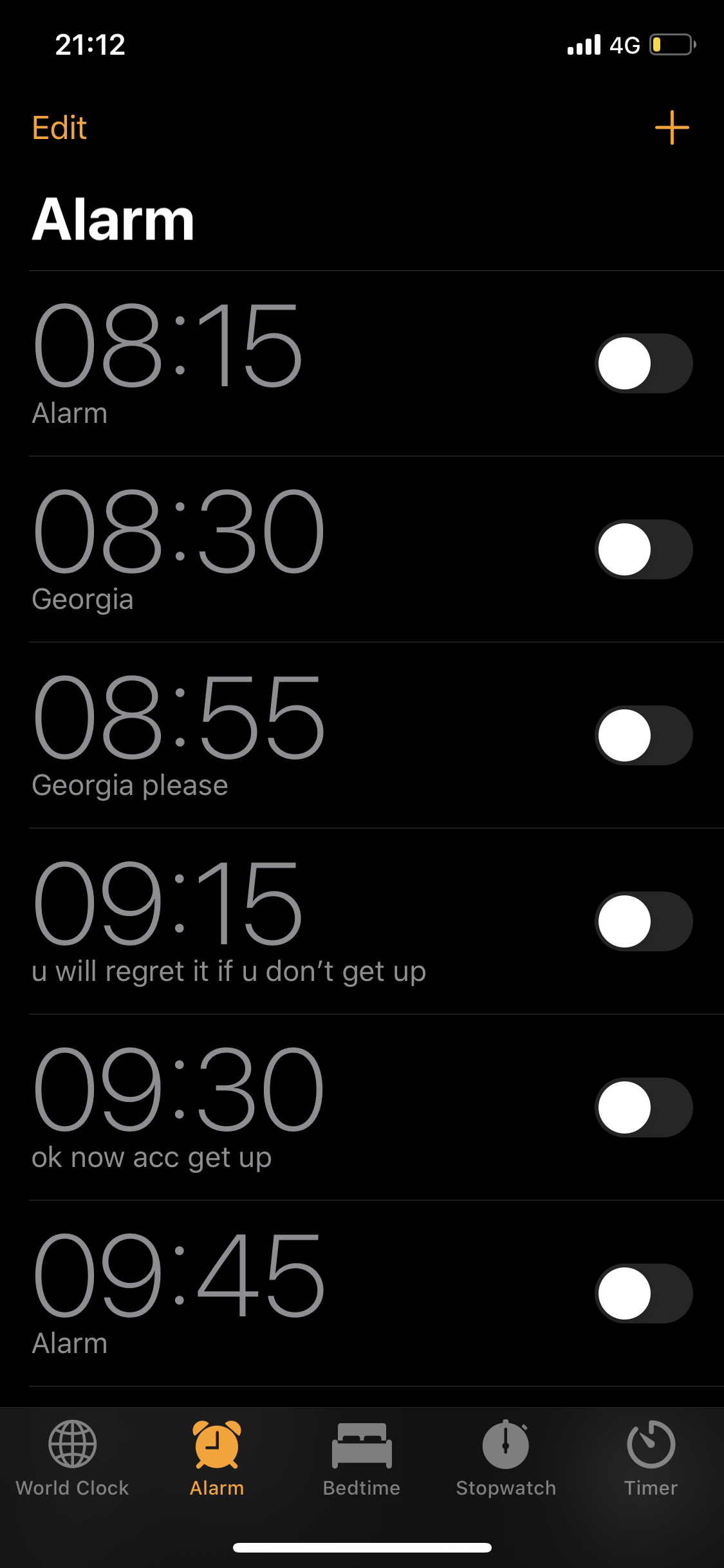The screenshot showcases an alarm-setting interface on a smartphone, displayed against a black background with a gray border at the bottom. The bottom border features five options in gray: World Clock, Alarm, Bedtime, Stopwatch, and Timer, with the Alarm option highlighted in orange, indicating that it is the current page. 

In the upper left-hand corner, the current time reads "21:12" in white text. The upper right-hand corner displays the phone's status: four of four signal bars, a 4G icon, and a nearly depleted battery icon in yellow. Just below, "Edit" appears in yellow on the left, and a yellow plus sign (+) is on the right, suggesting options to modify or add alarms.

The main screen lists several alarm settings, each with a gray toggle button on the right, all set to off:
1. "Alarm, 8:15"
2. "Alarm, 8:30" labeled "Georgia"
3. "Alarm, 8:55" labeled "Georgia, please"
4. "Alarm, 9:15" with the note "you will regret it if you don't get up"
5. "Alarm, 9:30" stating "okay, now ACC, get up"
6. "Alarm, 9:45" simply labeled as "Alarm"